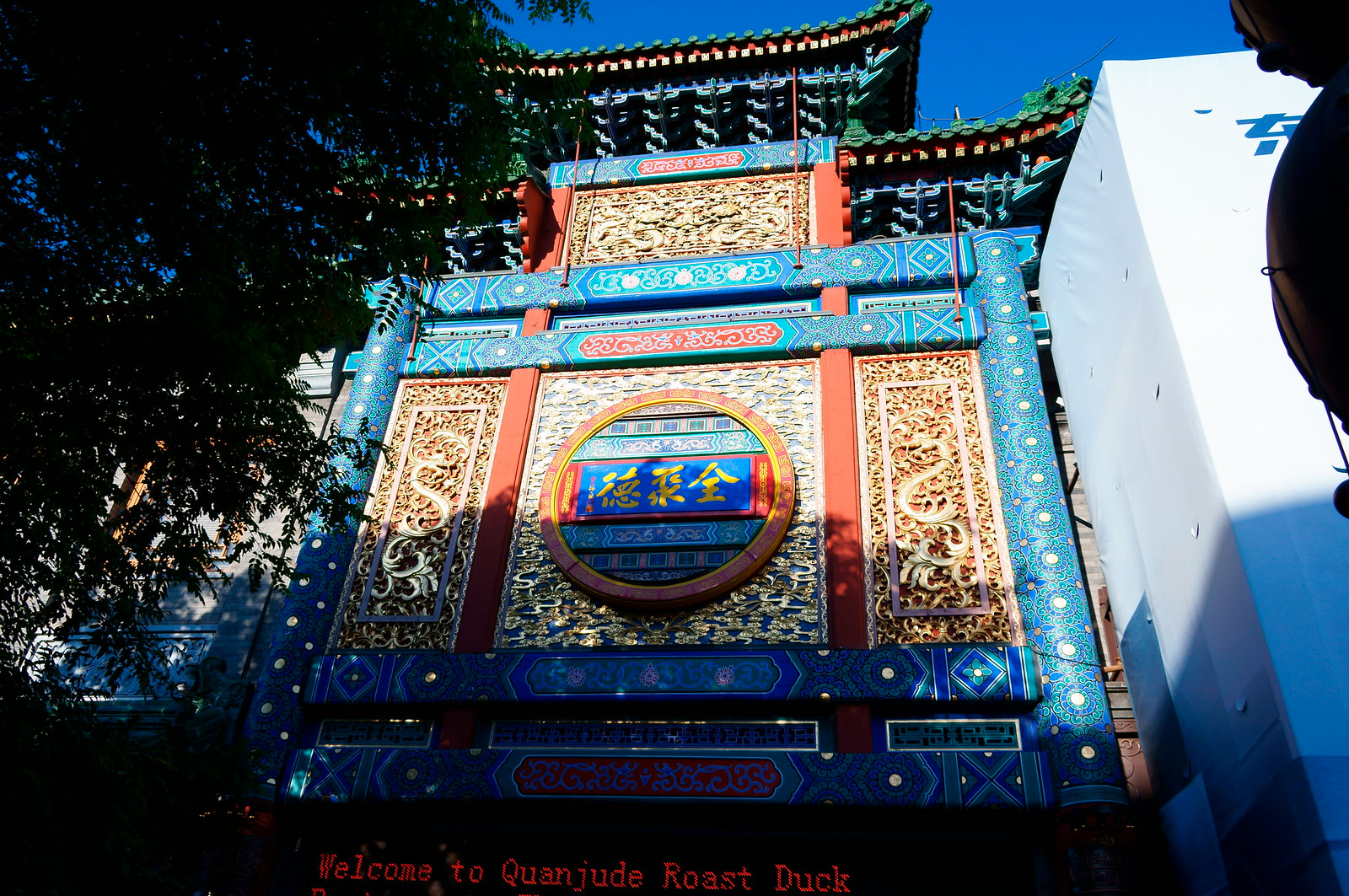The image captures the front of a very colorful, ornately decorated building resembling traditional East Asian architecture, likely Chinese. The building features blue trim accented with white dots, and red background areas with gray symbols. The centerpiece is a large circular design with a blue background, red edges, and yellow symbols. Adorned with intricate oriental decor, the structure includes tiered roofs and possibly a thatched section at the top, reminiscent of ancient buildings. At the bottom of the image, red letters on a black background read "Welcome to Kwanjude Roast Duck," indicating the name of the restaurant. The scene is framed against a clear blue sky, with tree branches and leaves partially obscuring the left side of the building, adding a touch of nature to the vibrant, cultural facade.